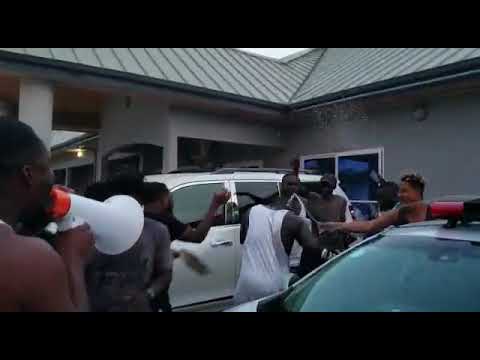The photograph captures a tense scene unfolding outside a building with a green slanted roof and gray walls. Set in a parking lot that could resemble a hotel or apartment complex, the image centers on a group of people engaged in an altercation between two cars—a white SUV in the background and another vehicle, likely gray, in the foreground. Among the seven to eight people present, most have their backs to the camera, while a few faces are visible. 

In the midst of the melee, four men of African descent appear to be arguing. One man, dressed in a long white sleeveless shirt, is crouching defensively, trying to shield his head. Nearby, a white man with blonde hair, possibly throwing a water bottle, adds to the chaotic scene. In the background, a black man holds up a bullhorn, possibly attempting to communicate or intervene, his face obscured by the device. Through these vivid details, the photograph conveys a moment of conflict and tension set against the mundane backdrop of everyday life.